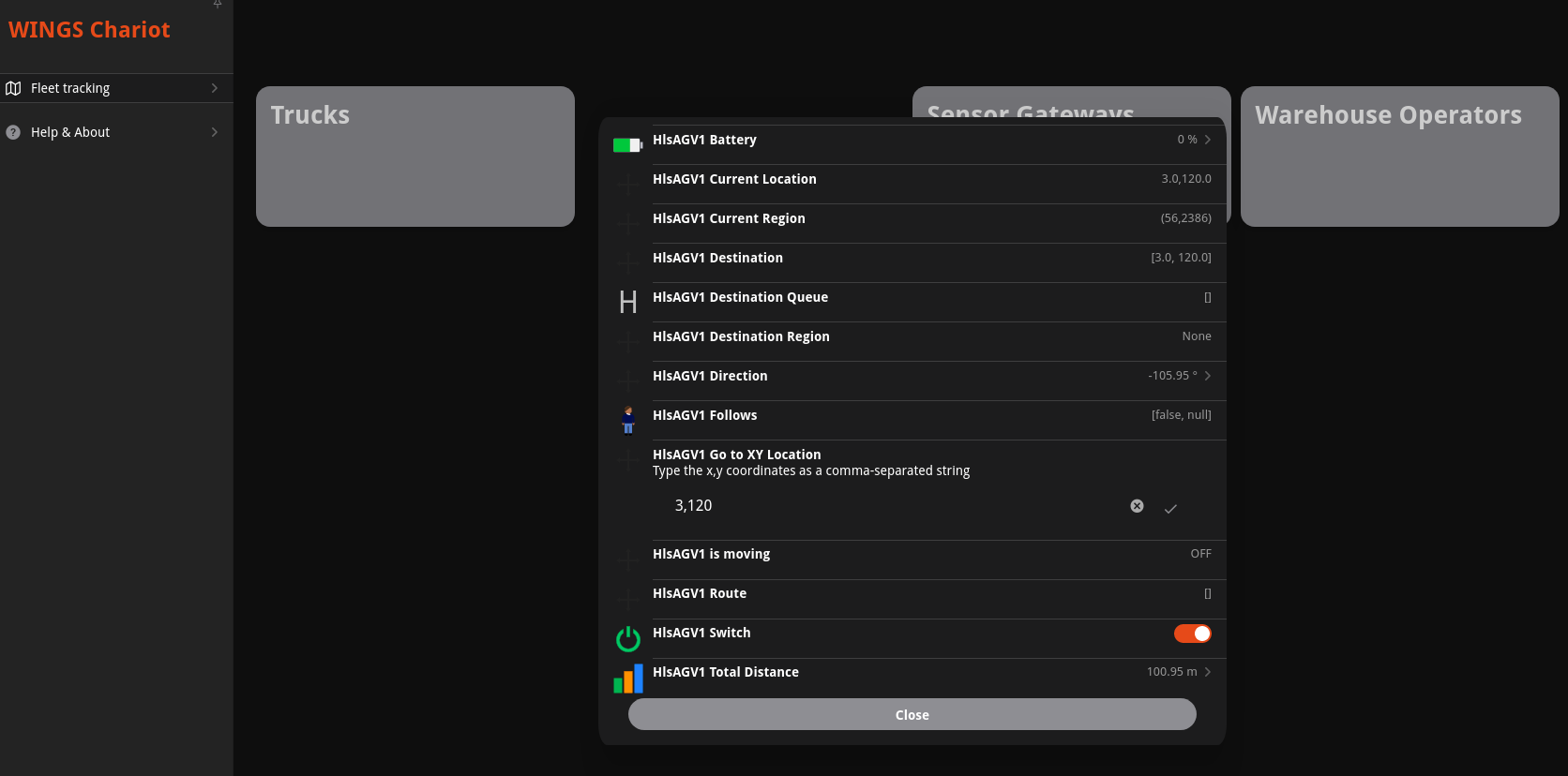The image prominently features the title "Wings Chariot" in bold, red text positioned at the top left corner. Directly beneath this title are two distinct categories. The first category, "Fleet Tracking," is accompanied by a small white icon of a mini truck to its left and a gray right-facing arrow to its right, creating a visual cue. Below this category lies the second one labeled "Help and About," which is indicated by a circular icon with a question mark on its left side and another gray right-facing arrow on its right.

The bottom left of the image contains a vast empty space extending downward. Central to the image is a prominent pop-up box with a black background, featuring a list of words in a square shape. Behind this pop-up, three boxes are discernible. The top left box is labeled "Trucks" in white text over a gray background. To its immediate right, there is another box titled "Sensor Gateways," also in white text on a gray background. Finally, at the top right, the box is marked "Warehouse Operators" in similar white text over a gray background, with all three background boxes appearing black.